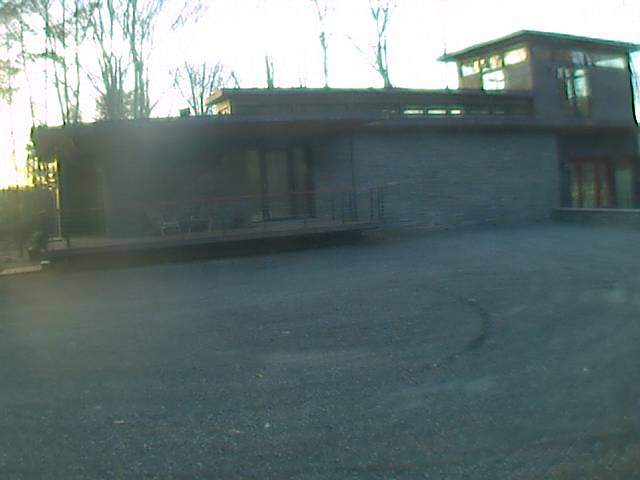In this sunlit but blurry photograph, we observe an outdoor scene captured during either sunrise or sunset, indicating a bright yellow or white washed sky along with a sunlit glare. The focal point is a two-story brick building, potentially a house, which exhibits both modern and slightly industrial characteristics. The structure, adorned with several unique window designs, including some that form a "T" shape on the upper level, appears to have a flat roof and a partially glass façade. There is a prominent red door on the right side of the first floor. Leading up to the house is a somewhat unkempt, dirt-streaked asphalt driveway that merges indistinguishably with a nearby parking lot. On the lower level, we note a deck equipped with some outdoor furniture and a glass door. The building, shaded in hues of gray and brown, subtly contrasts with its surroundings, blending almost seamlessly into the grayish-blue tones of the empty parking lot. Surrounding the house, particularly on the left side, stand several very thin, dark tree trunks, their black silhouettes stark against the well-lit horizon.